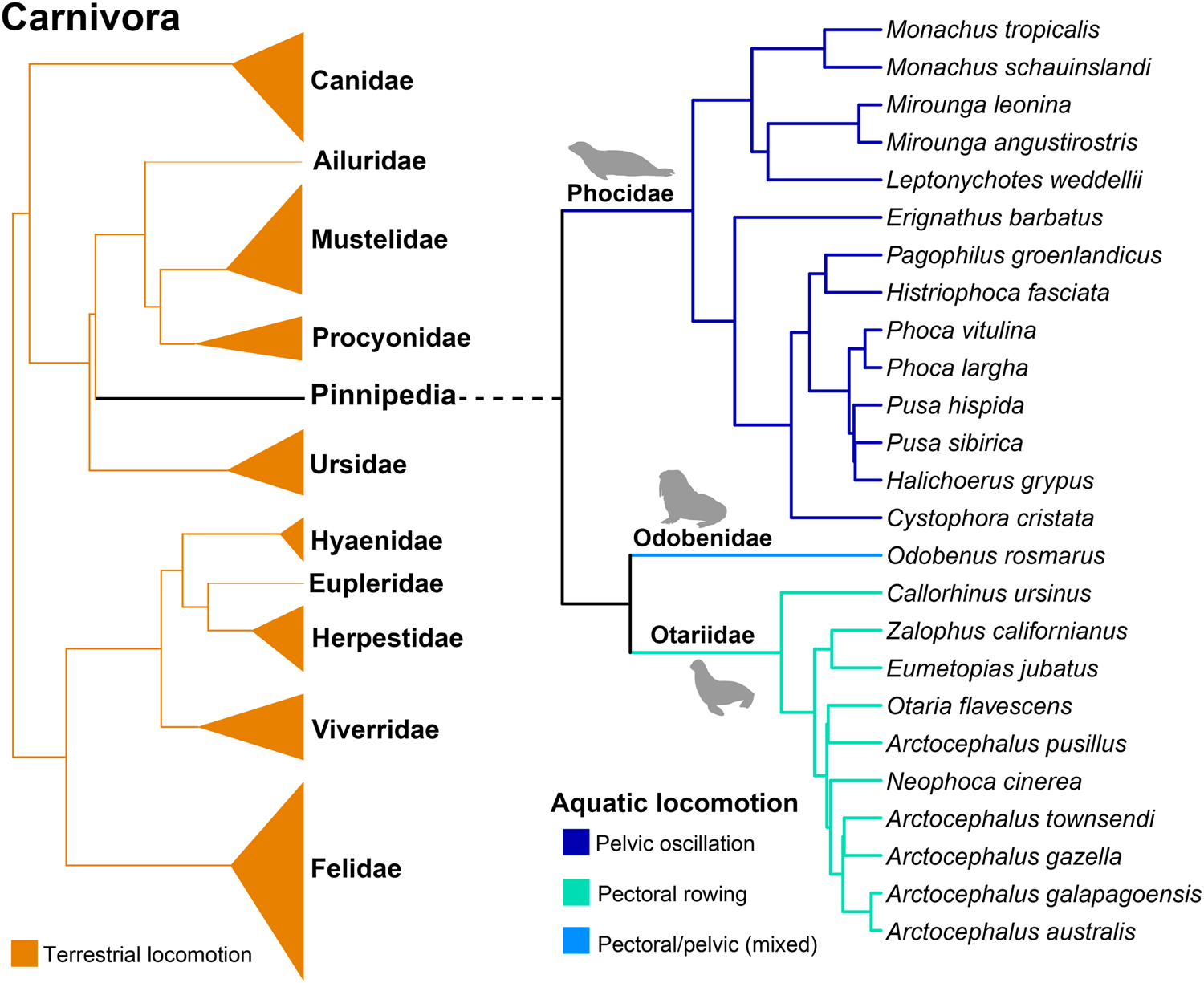The image is a detailed chart focusing on the Carnivora order, particularly exploring different families, genera, or species, with an emphasis on seals or sea lions. The chart uses a combination of orange shapes and lines on the left to represent the terrestrial locomotion of these animals, as indicated by a small orange square labeled "Terrestrial Locomotion" at the bottom. The diagram traces the Carnivora lineage and branches into various connected animal types, extending to possibly 10 or 11 on the left and over 20 on the right, depicted through blue connecting lines. Towards the right, it transitions into another chart under the category "Pinnipedia," which breaks down further into specific types of seals or related species, detailing their modes of aquatic locomotion. This section is color-coded, with categories such as "Pelvic Oscillation," "Pectoral Rowing," and "Pectoral/Pelvic Mixed," and includes images and scientific names of the depicted animal parts.